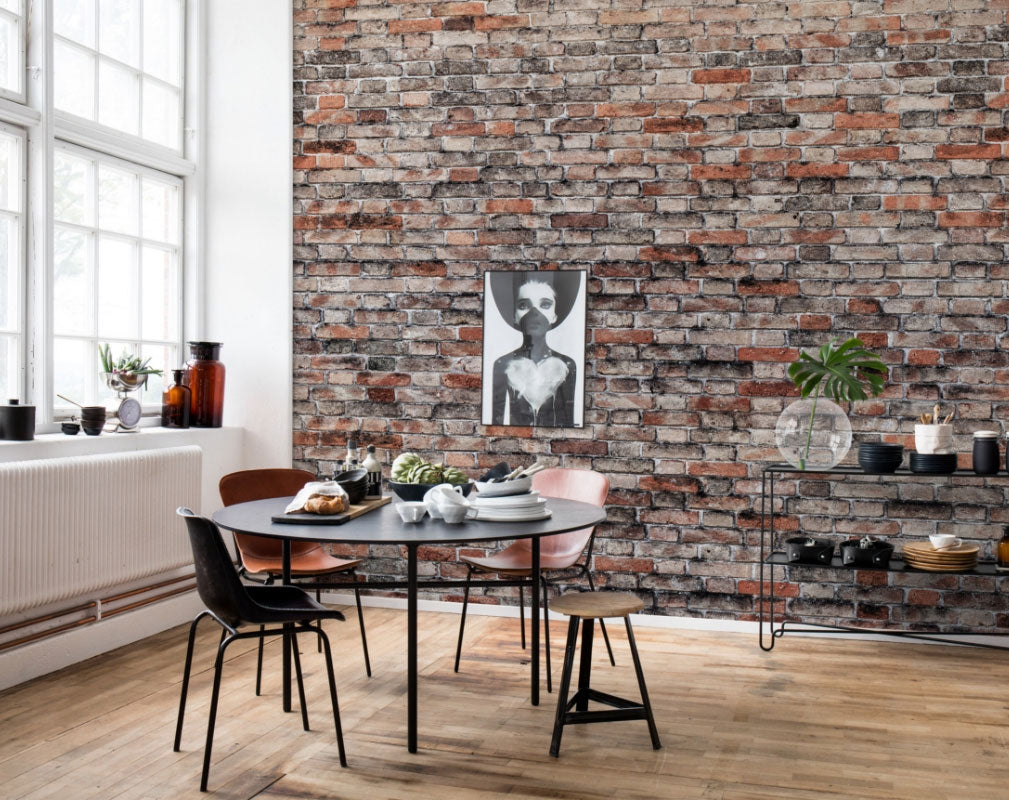The image showcases a modern dining area within a high-rise apartment or loft, featuring a mix of industrial and contemporary design elements. One wall is composed of exposed brick in shades of muted red, tan, gray, and white, adorned with a striking black-and-white photograph of a model with a large white heart painted on their chest. The adjacent wall is almost entirely made of windows, framed by a white half-wall that doubles as a shelf holding decorative items, including large amber glass jars, a kitchen scale, and bowls.

In front of the brick wall, a sleek wrought iron shelf displays a variety of objects: a plate, a cup filled with pencils, and a basket with a mug alongside other dark-colored dishware. This shelving unit complements the industrial flair of the space.

The foreground features a round dining table set for a meal, complete with white dinnerware, silverware, cups, and bowls. There is also a small wooden board with rolls and a bowl of fruit. The table is surrounded by modern chairs in a warm cognac color and includes a single stool, all situated on a light brown hardwood floor.

Natural sunlight streams in through the windows, illuminating the space and highlighting various decorative bottles and a small plant placed on the window ledge. An unobtrusive white radiator rests below the windows, blending seamlessly with the overall aesthetic.